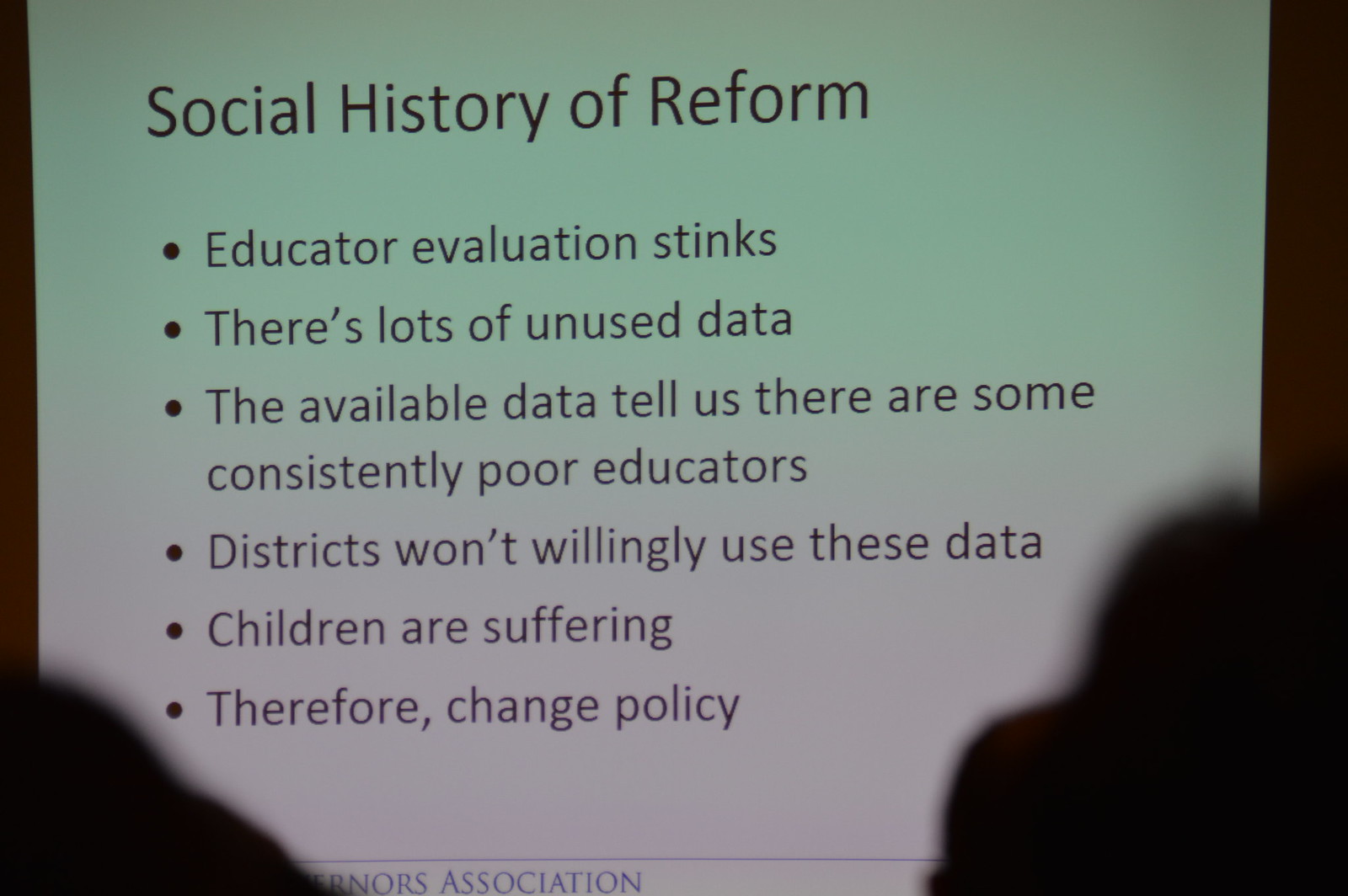The photograph captures a PowerPoint slide from a projected presentation, zoomed in and partially obscured by shadows on the bottom left and right sides, possibly from someone in the audience or objects in front of the screen. The slide has a white background with black text. At the top of the slide, the title "Social History of Reforms" is prominently displayed. Below the title are six bullet points:

1. Educator evaluation stinks.
2. There is a lot of unused data.
3. The available data tells us there are some consistently poor educators.
4. Districts won't willingly use these data.
5. Children are suffering.
6. Therefore, change policy.

Despite the detailed information, the text contains several grammatical errors. At the bottom of the slide, there is a mention of something "association" in blue text, though the full name is not clear due to the partial obstruction.